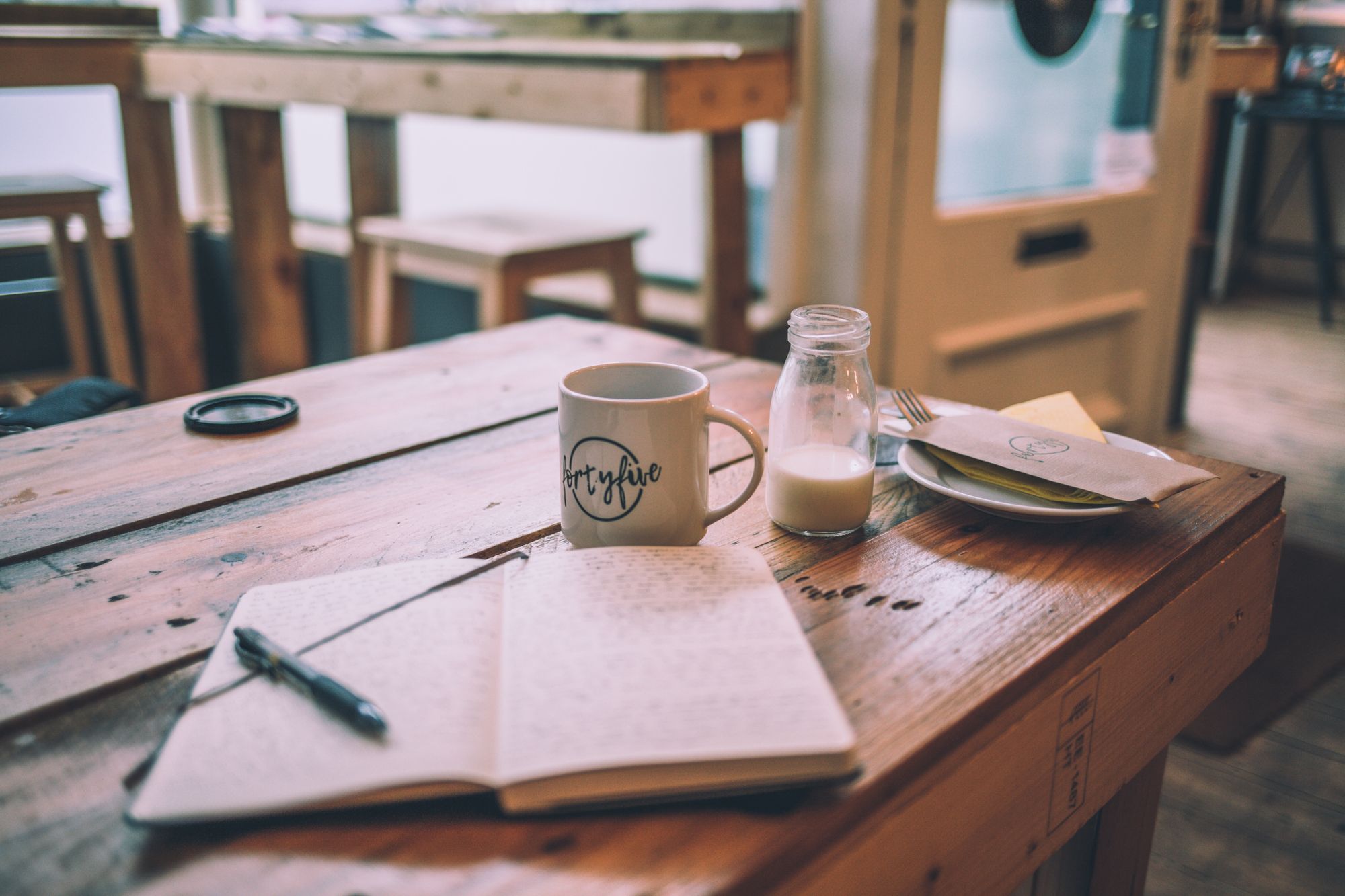The image depicts a rustic wooden coffee table adorned with various items. Central to the scene is an open journal with writing in black ink on both pages, accompanied by a black pen resting on it. To the left of the journal, there is a small glass jar, about a third full of milk. Nearby, a white coffee cup sits, featuring some text on its surface. Adjacent to the coffee cup is a plate holding a fork and what appears to be a brown napkin or wrapper. A drink blotter lies on the left side of the table, adding to the clutter. The background reveals an open door with a glass panel, leading to another room. This room houses another wooden table with stools tucked neatly underneath it, suggesting a cozy atmosphere, perhaps in a café or a coffee shop.